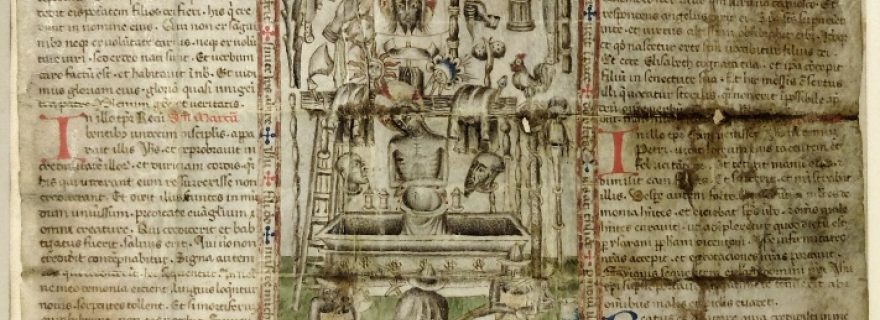The image appears to be a highly weathered and yellowed page from an ancient book or manuscript, possibly written in Latin. The page shows significant signs of wear, including wrinkles, blotches, and darkened folds, especially on the right side where it also seems slightly charred. There are two columns of elegantly written text, with some words highlighted in red for emphasis. In the center of the page, amidst the text, is a detailed illustration depicting a biblical scene. The main figure, likely Jesus Christ, is depicted rising from a coffin or tomb, looking malnourished with ribs visibly outlined. He appears to be wearing a white sheet around his waist. Behind him are various artifacts on shelves and a ladder to the left. The scene includes a cross, floating heads, a Sun, a moon, and other seemingly random objects, contributing to a surreal composition. The combination of text and imagery on this ancient, nearly burnt, and folded paper suggests a profound historical and possibly religious context.